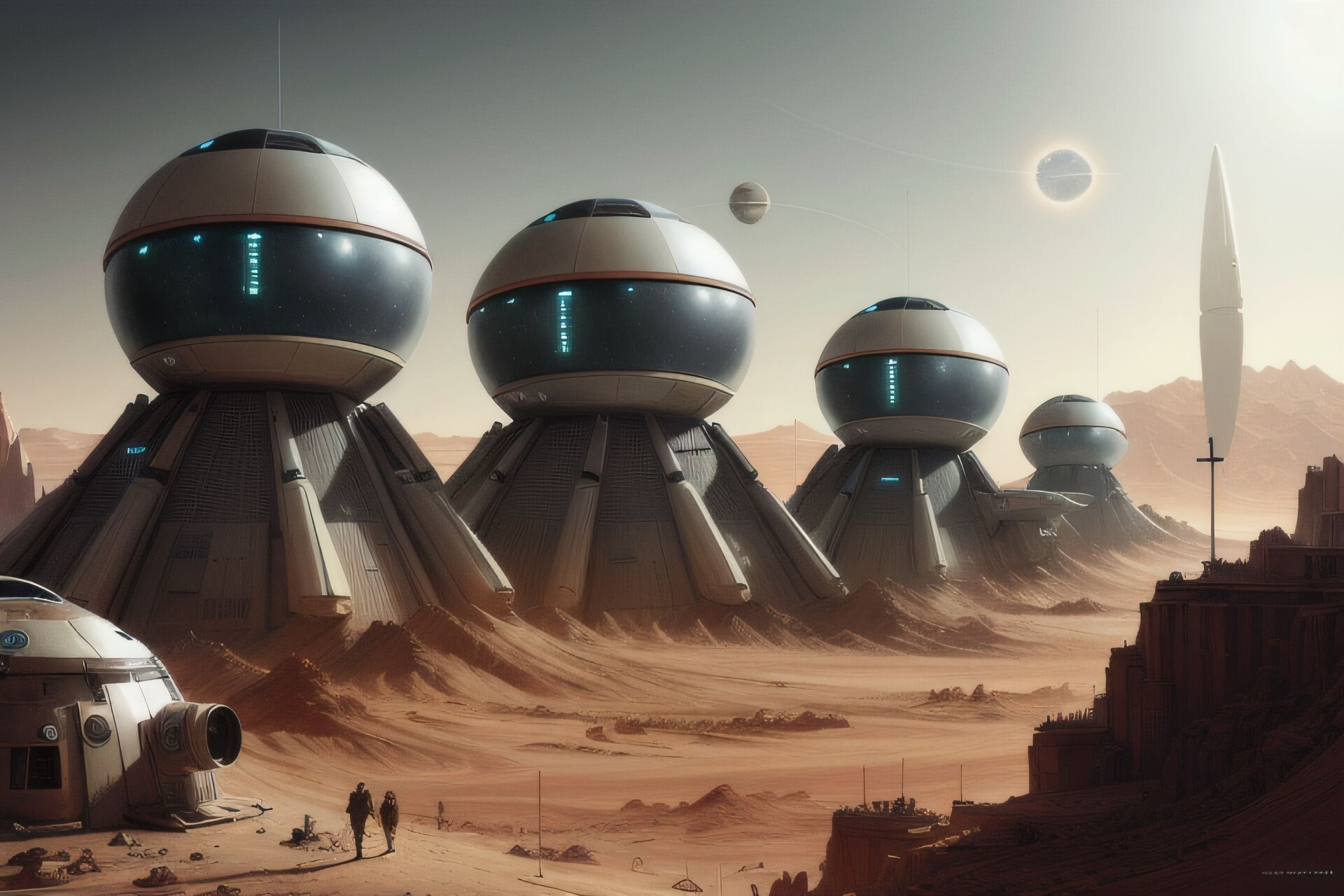This digital artwork depicts a futuristic civilization on a red sand desert planet. The sky is a somber gray, dominated by an eclipse in the upper right corner where a black sun, surrounded by a white ring, and an illuminated planet with a visible moon occupy the skyline. The sunlight emanates a stark white glow, casting shadows across the alien landscape.

The terrain below is characterized by red sand and desert mountain hills in the background, with a variety of architectural structures. On the left, a white dome-shaped home with a metal door marked by a white circle stands prominently. Toward the center and right, numerous pyramid-like buildings adorned with spherical tops rise from the surface, with a central feature resembling a volcano structure between four massive cylindrical edifices that resemble rockets or missiles supporting the sides. This central structure is topped with a white sphere that houses a see-through black window, glowing with blue symbols or lights inside.

Amidst these structures, two figures—one taller, possibly an adult, and a shorter figure, perhaps a teenager—navigate a series of stepped pathways shadowed by the towering edifices. Nearby, a cross stands out as a distinct marker on the landscape. Further right, there are rectangular buildings akin to those found on Earth, indicating a blend of alien and familiar elements in this advanced civilization.

Overall, the scene, marked by detailed and varied architecture, hints at a complex and technologically advanced society thriving on an extraterrestrial world, under an otherworldly sky punctuated by cosmic phenomena.